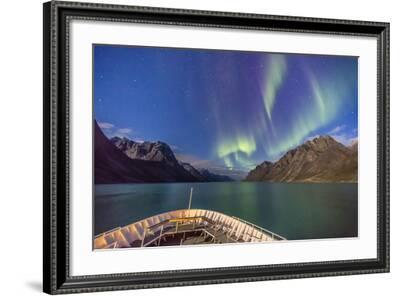The image depicts a framed photograph featuring a serene lakeside scene under a mesmerizing night sky. The black rectangular frame, adorned with subtle decorations around the edge, encases the photograph, with a white matting providing contrast. The main artwork within the frame portrays calm, greenish-blue water reflecting the vivid sky above. In the foreground, the tan-colored tip of a boat is visible, adding a sense of adventure. The tranquil water leads the eye to the rugged, dark gray mountains that stretch horizontally across the center. Above the mountains, the sky boasts an ethereal display of the Northern Lights, predominantly showcasing hues of yellow and purple with hints of green and blue, punctuated by small white dots resembling stars. The photograph is slightly tilted to the right, adding a dynamic angle to the composition.